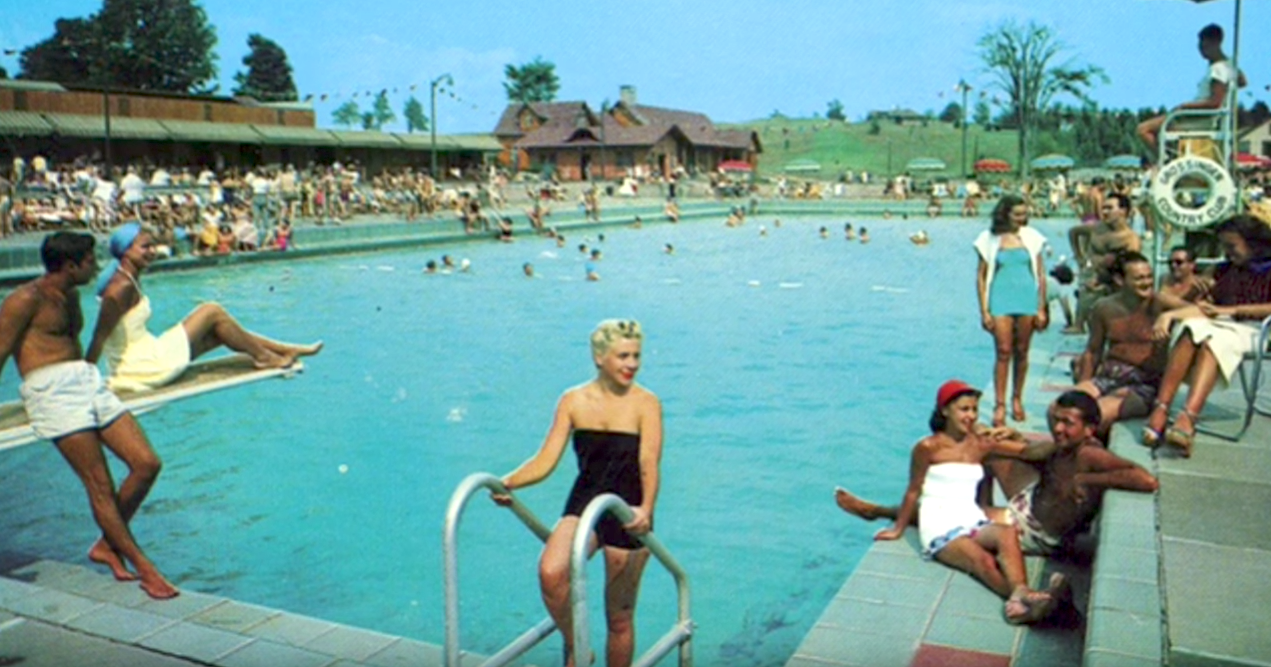This 1950s photograph captures a bustling summer scene at an enormous, rectangular community swimming pool, almost pond-like in size. The focal point is a blonde woman with a Marilyn Monroe-like appearance, dressed in a black bathing suit, as she climbs out of the pool using metal rails at the bottom center of the image. Surrounding her, the edges of the pool are brimming with people, reminiscent of a stadium's density, creating an almost collage-like effect.

To her left, a diving board extends over the water, where a man in white shorts leans against it and a woman in a white sundress with blue headwear sits on it. The company around the pool is diverse, with numerous people of different backgrounds sitting, lying, talking, and swimming in the deep end. There is a lifeguard perched above the crowd on the right-hand side.

In the background, the left side features a large building, possibly a country club, and on the right, a long, narrow roofed structure shelters more people. Trees, grass, and strung-up decorations add to the lively ambiance. Streetlights and other structures further frame the scene, emphasizing the community's vibrant life.